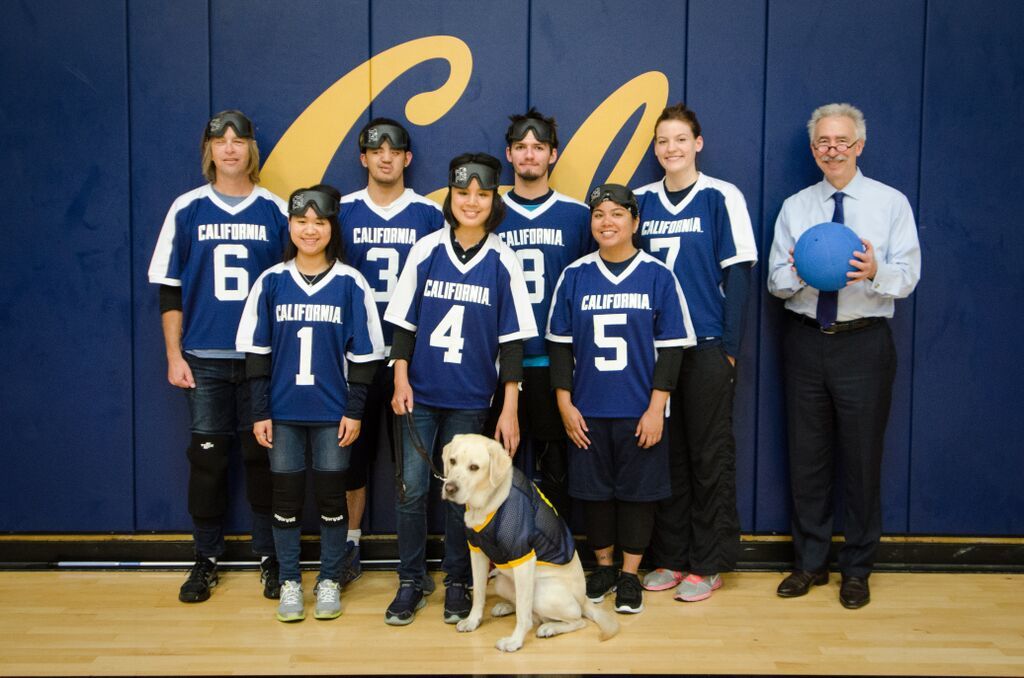In the photo, a group of seven kids, seemingly part of a dodgeball team, stand in front of a padded, blue wall adorned with the yellow word "Cal." They wear blue jerseys with bold white text reading "California" and stripes down the sleeves. Each jersey is numbered from 1 to 7. The team members, comprising both males and females, have heavy goggles perched above their eyes and some are equipped with knee pads. In the front row sits a golden Labrador, also in a blue jersey with a yellow collar. To the right of the group stands an older gentleman, likely the coach, dressed in black pants, a white shirt with a blue necktie, and holding a blue ball. The setting appears to be a gymnasium.